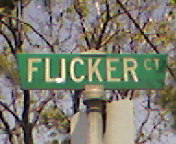This is a close-up color photograph of a green street sign against a backdrop of a blue sky and tree branches. The narrow rectangular sign is prominently featured, with white lettering that is meant to spell "Flicker Ct." However, someone has defaced the sign by connecting the letter "L" and the letter "I," resulting in an altered version that now reads "Fucker Ct." The juxtaposition of the serene natural background with the vandalized sign creates an unintended humorous effect.